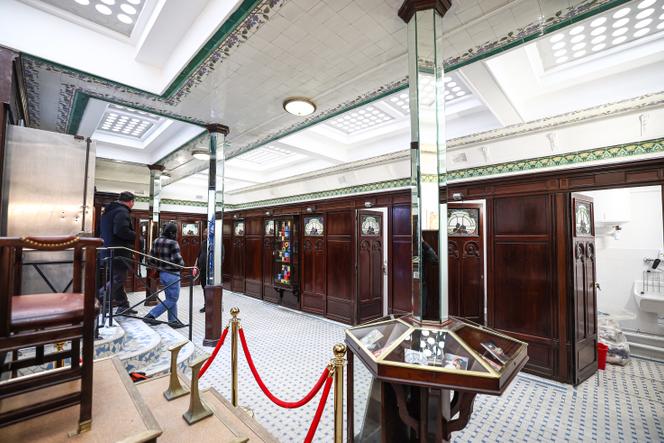The photo depicts the spacious lobby of a building that bears a resemblance to a museum or a high-end bathroom facility. On the left side of the image, two individuals are walking down a set of stairs. They appear to have just entered the room, with one person wearing a coat and the other in a flannel shirt with blue jeans. They are not the focal point of the image. 

The room has a series of wooden doors lined up along its walls, each door featuring a glass pane at the top and intricate patterns. Some doors seem to open into separate bathroom stalls, potentially containing amenities like urinals, saunas, and showers. The bathroom areas are said to be predominantly white inside.

In the background, a seating area is visible, which is cordoned off by a red velvet rope with gold stanchions, possibly indicating an exhibit or restricted section. A large column, with various objects encased at its base, stands nearby. A tall stainless steel fridge can also be seen to the left of the individuals. The ceiling is adorned with various patterns and lit by several lights, contributing to the room's bright and open ambiance. The overall appearance of the image is realistic and detailed, suggesting that it is indeed a photograph.